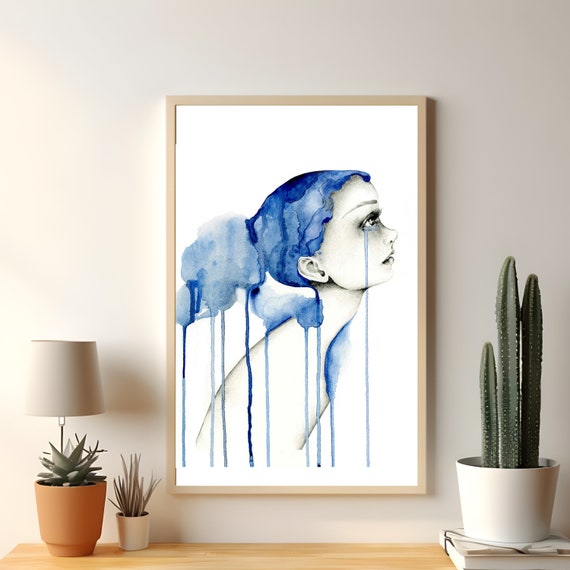The image is a square-format color photograph capturing a well-composed interior scene. The focal point is a vertical, light wood-framed painting hanging on a beige wall above a light wood side table. The painting depicts a young woman in profile, viewed from the side and facing upward to the right. Her blue hair is styled in a bun, with blue watercolor dripping from both her hair and eyes, suggesting she is crying. The background of the painting is white, adding to the melancholic effect. Below the painting, the side table features a small lamp with a beige shade on the left, a terracotta planter with an aloe vera plant, and a small grassy-looking plant in a white container. To the right, there's a green cactus in a white vase sitting on top of a book. The arrangement of these elements creates a harmonious and detailed interior scene, with the emotionally evocative painting as the central piece.